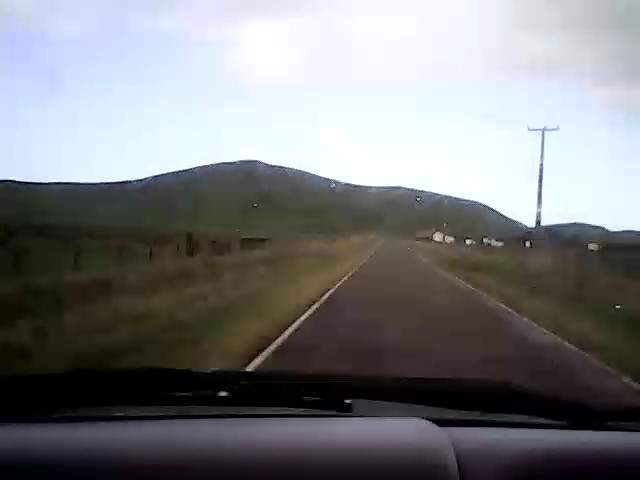The horizontal image captures the view from inside a vehicle traveling down a single-lane paved road in a scenic rural area. The dashboard is visible, showing a dark hood with a gray or light purple interior. The road, marked with a white line on the left edge, stretches ahead towards a small village characterized by white buildings with dark brown roofs. 

The landscape features relatively flat grasslands on either side, framed by vineyards and possibly a fence to the left. The backdrop consists of hills and mountains with several ridges that slope down toward the village. A very tall utility pole stands in the distance on the right side, although no power lines are visible. The photograph is somewhat blurry, giving it a low-resolution appearance rather than a motion-blur effect.

The sky is partially cloudy with the sun peeking from behind, casting a fair amount of light despite the car's headlights being on. Trees are visible in the background, most noticeably on the opposite side of the road.